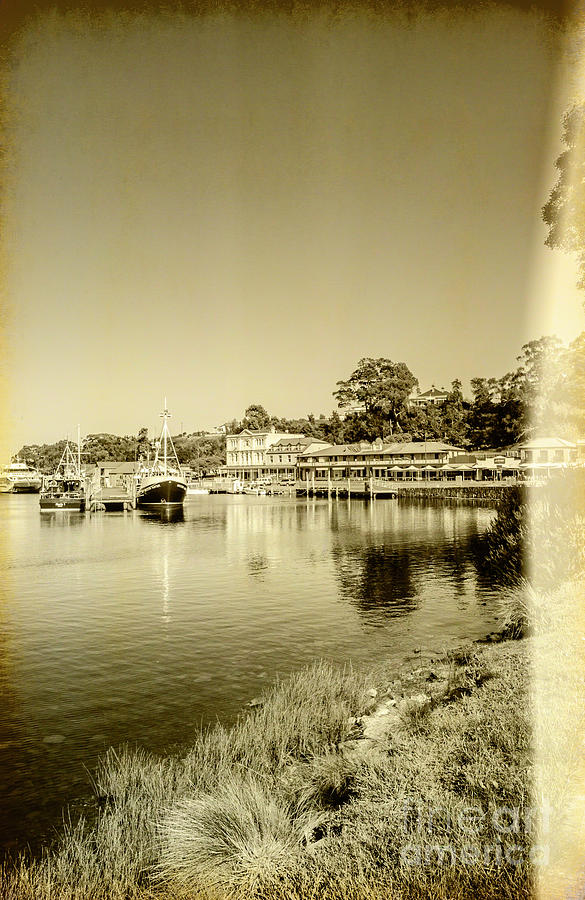This vintage photograph, rendered in sepia tones with hints of yellow and brown, captures a serene marina scene. The image is marked with age, evident from the browned edges and a vertical sun glare running along the right side. The sky is clear, and a gently sloping grassy area frames the bottom right corner, ascending from left to right.

In the background, a dense tree line forms a natural border behind the marina and its buildings. Two structures sit on the hillside next to the tree line. The shore stretches along the midsection of the photograph, lined with buildings to the right, where cars and people are visible. A dock juts out toward the water from the central building, adding depth to the scene.

Three medium-sized boats float on the calm waters. The boat closest to the right, notable for its large bottom, contrasts with the two flat-bottomed boats to the left. There are no sails deployed on any of the boats. The clear reflections of the trees dance on the water’s surface, enhancing the image's tranquility. A faded, unreadable text earmarks the bottom right side, adding a mysterious touch to this evocative snapshot from the past.